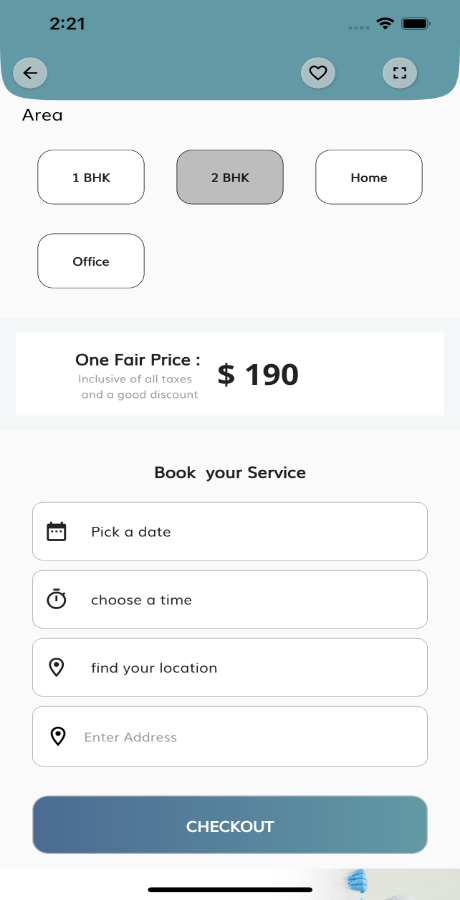Screenshot of Service Booking Interface: 

The image is a screenshot of a service booking interface, with a visually appealing layout highlighted by a clean, blue color scheme. At the top of the screen, there's a status bar displaying essential information such as the remaining battery life. To the left, an arrow labeled "Area" suggests navigation, though its exact function is unclear. Adjacent to it are icons including a heart and a button to expand the page view. The interface features four selectable blocks labeled "1BHK" and "2BHK," with the "2BHK" option highlighted in gray, indicating it is currently selected. 

Central to the layout is the service description and pricing, stating "One fare price, $190." Additional instructions prompt users to "Book your service," guiding them through steps like picking a date, choosing a time, finding their location, entering their address, and checking out. Despite the clear procedural steps, the specific nature of the service remains unspecified.